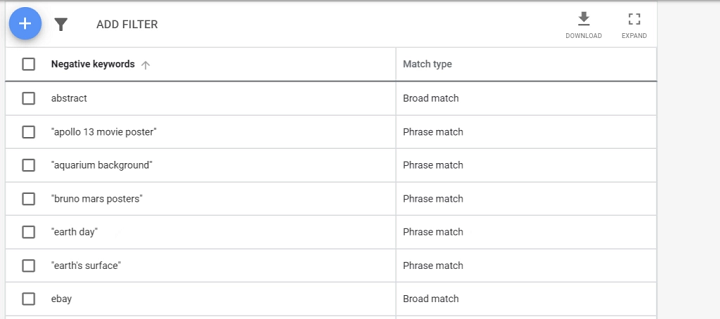Detailed Image Description: 

The screenshot features a user interface with a gray background. At the top, there is a blue circle containing a white plus sign, accompanied by an "Add Filter" label. Below this section, there is a gray filter icon alongside a download symbol, indicating features for applying and downloading filters. There are options labeled "Download" and "Expand", both represented by square icons.

The interface prominently includes a series of checkboxes next to various navigation keywords. An up arrow is displayed to denote sorting or prioritization functionality. Keywords listed include: 

- **"Apollo 13 movie poster"** with a **Phrase Match** filter
- **"Aquarium background"** with a **Phrase Match** filter
- **"Bruno Mars posters"** with a **Phrase Match** filter
- **"Earth Day"** with a **Phrase Match** filter
- **"Earth's surface"** with a **Phrase Match** filter
- **"eBay"** with a **Broad Match** filter

These keywords and their respective match types suggest a search or filtering mechanism refined by specific matching criteria.